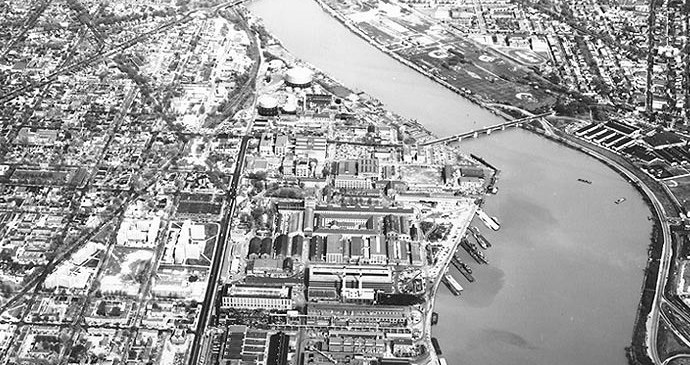This black and white, aerial photograph offers a striking, historical view of an industrial city, potentially reminiscent of early 1900s New York City or Chicago. Dominating the scene, a wide river runs diagonally from the bottom right to the upper left, narrowing as it progresses. It is spanned by a prominent bridge near the center of the image, connecting the two distinct sections of the city. On both sides of the river, dense arrays of roadways form a grid system crisscrossing between numerous large buildings and industrial structures, including apparent cisterns and a partially visible metal tower on the right. The left side of the river showcases slightly more land, while scattered grassy areas add minor patches of greenery to the urban landscape. At the bottom of the river, various boats and docks are visible, reinforcing the impression of a bustling harbor area.